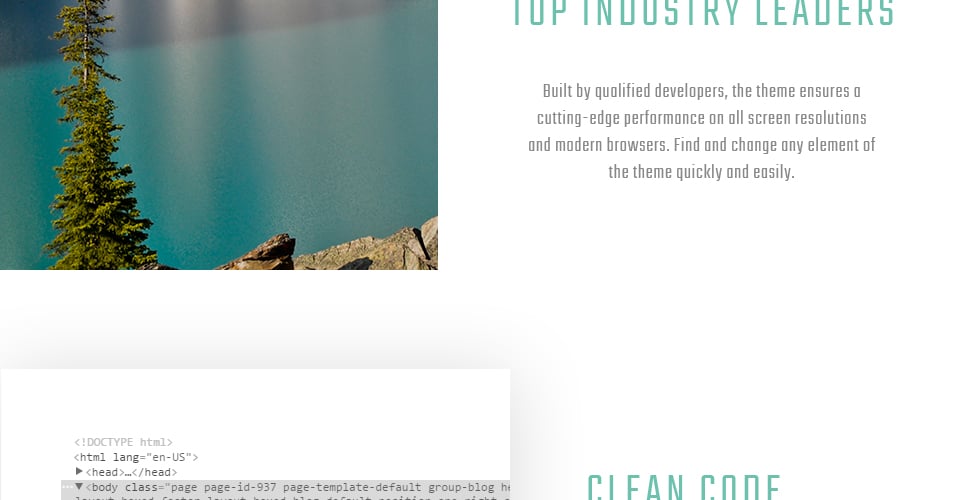**Detailed Caption:**

This screenshot captures a segment of a webpage designed for software development. The layout is divided into two main content sections, each partially cut off.

The top section features a two-column format. The left column displays an image with the top view of an evergreen tree situated near a body of water. The upper left corner of the image reveals the tree's foliage against a backdrop of water, which shifts from a very dark shade at the top to a lighter, almost teal-blue hue dominating the middle of the image. A small rocky area appears in the bottom right corner.

To the right of the image, the second column contains textual content. The headline reads "Top Industry Leaders," although the top portion of each letter is truncated, making the 'T' resemble an 'I' and the 'S' appear incomplete. Below the headline, a descriptive paragraph follows, reading: "Built by qualified developers, the theme ensures a cutting-edge performance on all screen resolutions in modern browsers. Find and change any element of the theme quickly and easily." This text is center-justified and spans four lines.

The bottom section mirrors the two-column layout of the top section. The left column shows a code snippet with a white background, indicating HTML content. The visible part of the snippet reads:
```
<!DOCTYPE html>
<html lang="en-US">
  <head>
    <title>HTML Style</title>
  </head>
  <body class="page-id-937 page-template-default group-blog">
...
```
The snippet appears to be highlighted in a dark gray shade and is cut off at the end. On the right, a headline in green reads "Clean Code," although the bottom portions of each letter are missing.

Overall, this webpage blends visual elements with technical content, catering to an audience interested in software development and performance optimization.